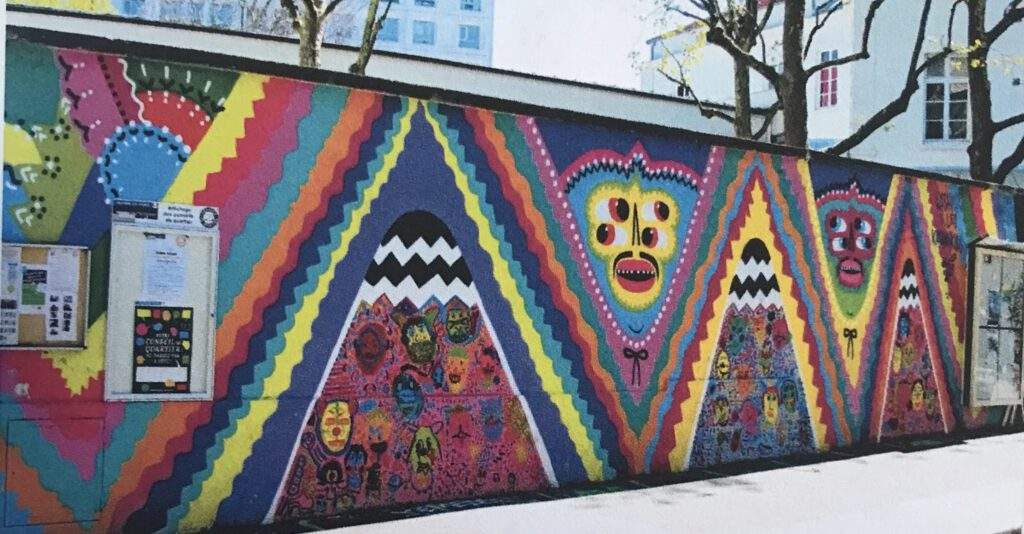The vibrant outdoor mural features an array of vivid colors, predominantly greens, blues, reds, yellows, and oranges, creating a psychedelic ambiance on what appears to be a dividing wall along a sidewalk. This mural is rich in detailed, intricate patterns, including diagonal rainbow-colored stripes, zigzag lines, and triangular shapes. Dominating the artwork are various human faces with distinctive features, such as two pairs of eyes—some gazing in different directions—with a mix of yellow, blue, and red hues. Some faces resemble African mascots, further adding to the mural's cultural depth.

In addition to the colorful artwork, there are several functional elements integrated into the scene. On the left side of the mural, there is a metallic box with buttons, predominantly in red, yellow, and green, accompanied by small, unreadable white notices. Nearby, another smaller white rectangle also features notes. Above the mural, one can see trees and distant buildings, including a tall structure with visible windows and a red curtain in one of them. The mural is set against the backdrop of a bright sky, with occasional glimpses of what could be an apartment complex peeking from the upper left corner of the image.